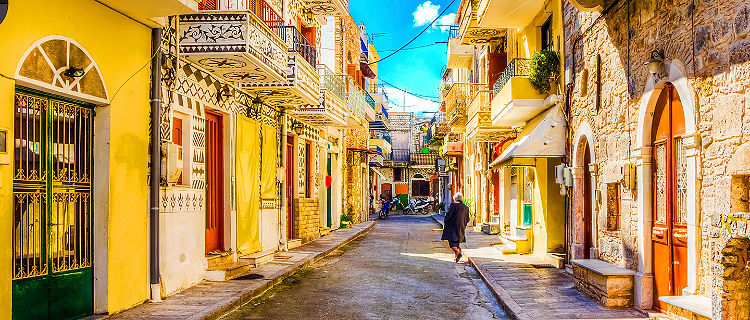The image depicts a vibrant urban scene in what appears to be a European or Asian city, with a narrow street flanked by sidewalks on either side. The sky above is a bright blue adorned with white, fluffy clouds, casting ample sunlight across the scene. The buildings lining the street are bathed in natural light, featuring predominantly yellow and warm beige exteriors. These structures showcase a mix of architectural details, including numerous doors, balconies with railings, and varied color palettes that include white, orange, and brick. Far in the distance, a building with a prominent orange facade stands out. The street scene includes a few motorcycles parked against the buildings, adding a touch of everyday life. A woman with gray hair, dressed in a long jacket or black shawl, is seen crossing from the sidewalk onto the street, further emphasizing the tranquility and minimal bustle of this picturesque setting.